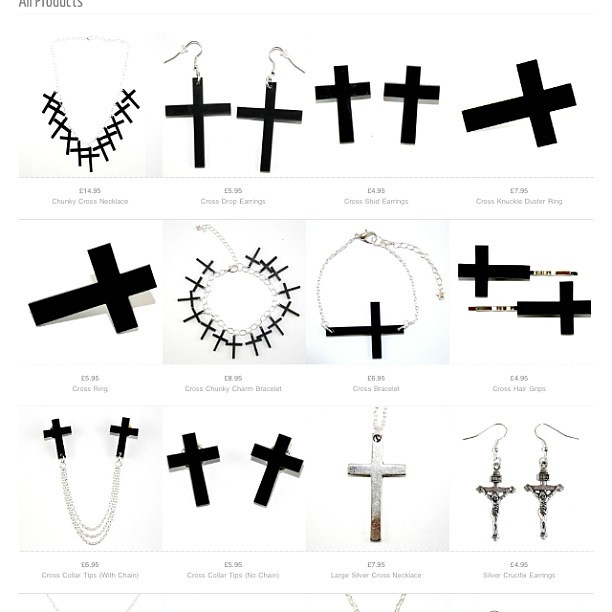In this image, we see a collection of jewelry pieces, all featuring cross designs, with prices listed in pounds and pence. The top left corner of the image has partially cut-off text that likely reads "all products." The displayed items are arranged in three rows and consist of 12 main images, although 16 were originally intended, and four are cut off at the bottom.

The first row features a chunky silver necklace adorned with multiple black crosses priced at £14.95. Next are two pairs of black cross earrings: one pair with hook-style attachments priced at £5.95 and another pair of large cross studs priced at £4.95. The fourth item is a cross knuckle duster ring with a single horizontal black cross, priced at £7.95.

In the second row, there's a black cross ring priced at £5.95, followed by a chunky charm bracelet featuring several black crosses, priced at £2.95. The next item is another bracelet with a single black cross laid horizontally, priced at £5.95. Completing the second row are two black cross hair grips with silvery tips at the bottom, priced at £4.95.

The third row begins with a set of cross collar tips featuring two black crosses and long dangling chains, priced at £5.95. Another pair of cross collar tips without chains is priced at £5.95. Additionally, there is a large silver cross necklace with a brownish bottom priced at £7.95. The final item is a set of silver crucifix earrings featuring a Jesus figure on each, priced at £5.95. All the crosses in the image are black, square, and carry a chunky design.